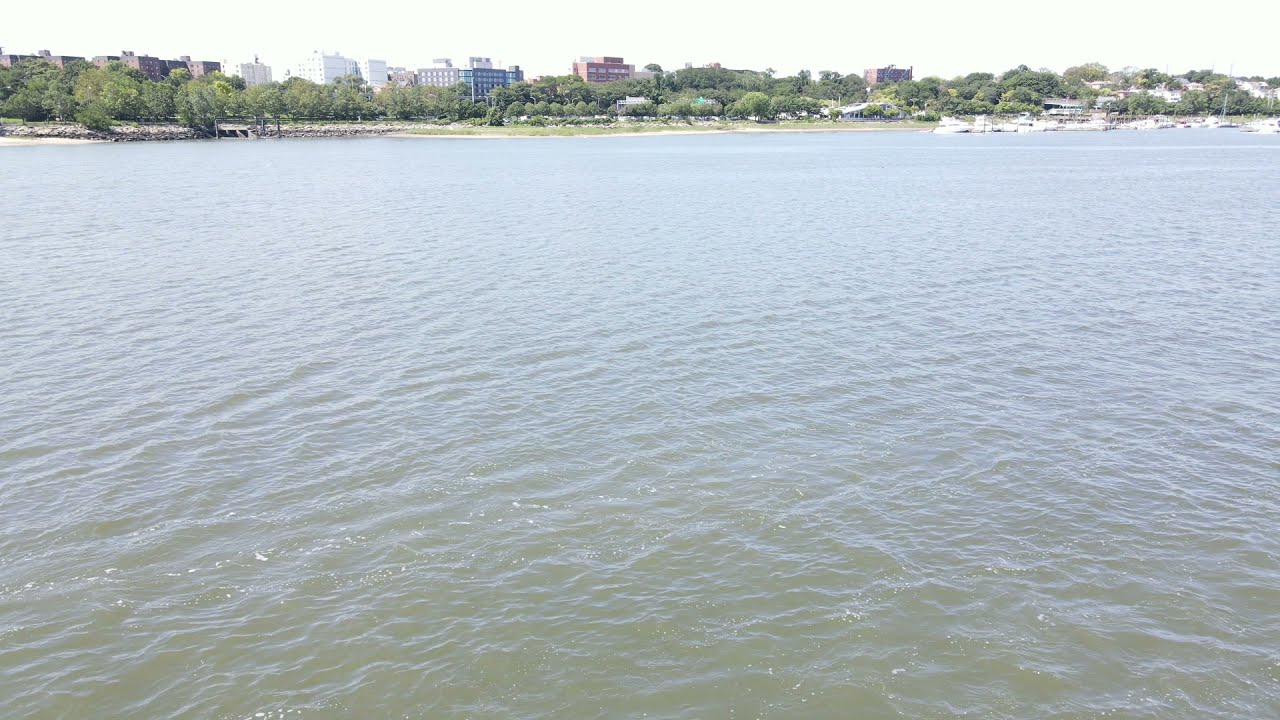The image captures a calm, wide river with murky green waters and slight ripples. The photograph is taken from a boat-level perspective, giving the view of the water and the cityscape beyond. The scene encompasses a sprawling river occupying most of the frame, gradually leading to a city settled on its perimeter. On the left side, there are clusters of tall buildings, eight to ten stories high, including a prominent blue office building to the left of a red brick structure. Toward the right, a boat harbor hosts an array of smaller boats and sailboats near the edge of the water. Nestled behind the harbor is a walking path bordered by lush green trees. The background features a mix of greenery and urban architecture, highlighting an industrial or commercial district rather than residential. The sky above is predominantly white, devoid of clouds, enhancing the contrast between the serene water and the structured city backdrop. Rocks where the water meets the land punctuate the shoreline, contributing to the tranquil yet dynamic composition of the image.